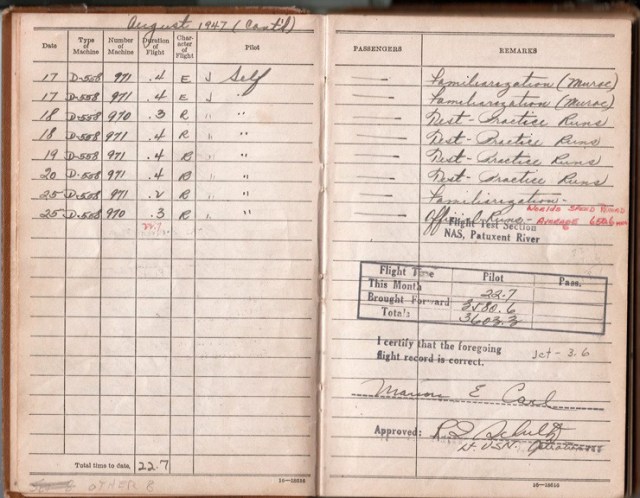The image depicts an open flight logbook from August 1947, showing detailed records of flights conducted during that month. On the left page, there are six vertical columns labeled: Date, Type of Machine, Number of Machine, Duration of Flight, Character of Flight, and Pilot. The right page features two columns: Passengers and Remarks. Each column provides specific entries, with the dates ranging from August 17th to August 25th, noting details such as the aircraft identification D-508 and D-558, and flight durations. The character of the flights is marked with letters like 'E' and 'R', and the pilot column repeatedly lists "J SELF."

The remarks section includes handwritten notes like "familiarization (MURAC)," "test-practice runs," and an official stamp stating "Flight Test Station NAS Patuxent River," indicating the location as the Naval Air Station Patuxent River in Maryland, not Virginia as originally thought. Signatures and stamps are found below the log entries, certifying the accuracy of the records and featuring the names Marion E. Carl and Lieutenant Schultz, USN. Additionally, a cumulative flight time is recorded as 3603.3 hours. The pages display a vintage look with a pinkish or light brown tint consistent with an old document, confirming its age of approximately 76 years.